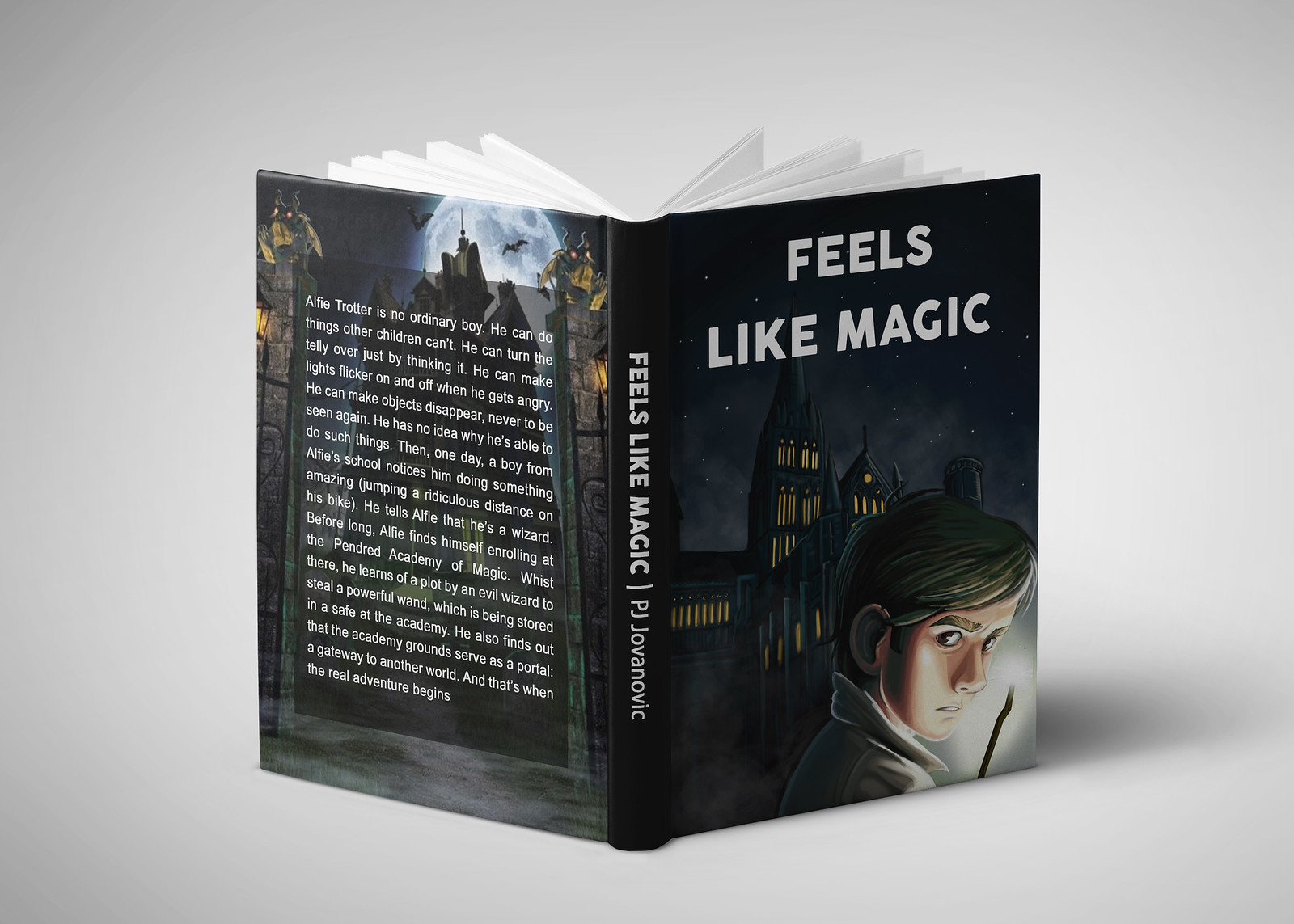The image depicts a hardcover book standing upright on a white, grayish-white background. The book's front cover, which is dark gray and black, displays the title "Feels Like Magic" in white font, with "Feels" on the first line and "Like Magic" on the second. The spine of the book also reads "Feels Like Magic" by P.J. Jovanovich. On the front cover, there's an illustration of a person with short hair and thick eyebrows, wearing a white jacket and looking over their shoulder with a frightened expression. A stick emitting light from its tip is near them. Behind the person is a tall, old, and scary-looking building with lit yellow windows, evoking a nighttime scene. The back cover also features this eerie house, with additional details like a moon and bats flying around, along with a descriptive paragraph about the book. The synopsis reveals that a boy named Alfie is noticed by a classmate for performing an extraordinary bike jump, leading to the revelation that Alfie is a wizard. Alfie enrolls at the Pendret Academy of Magic, where he uncovers an evil wizard's plot to steal a powerful wand and learns that the academy grounds serve as a portal to another world.